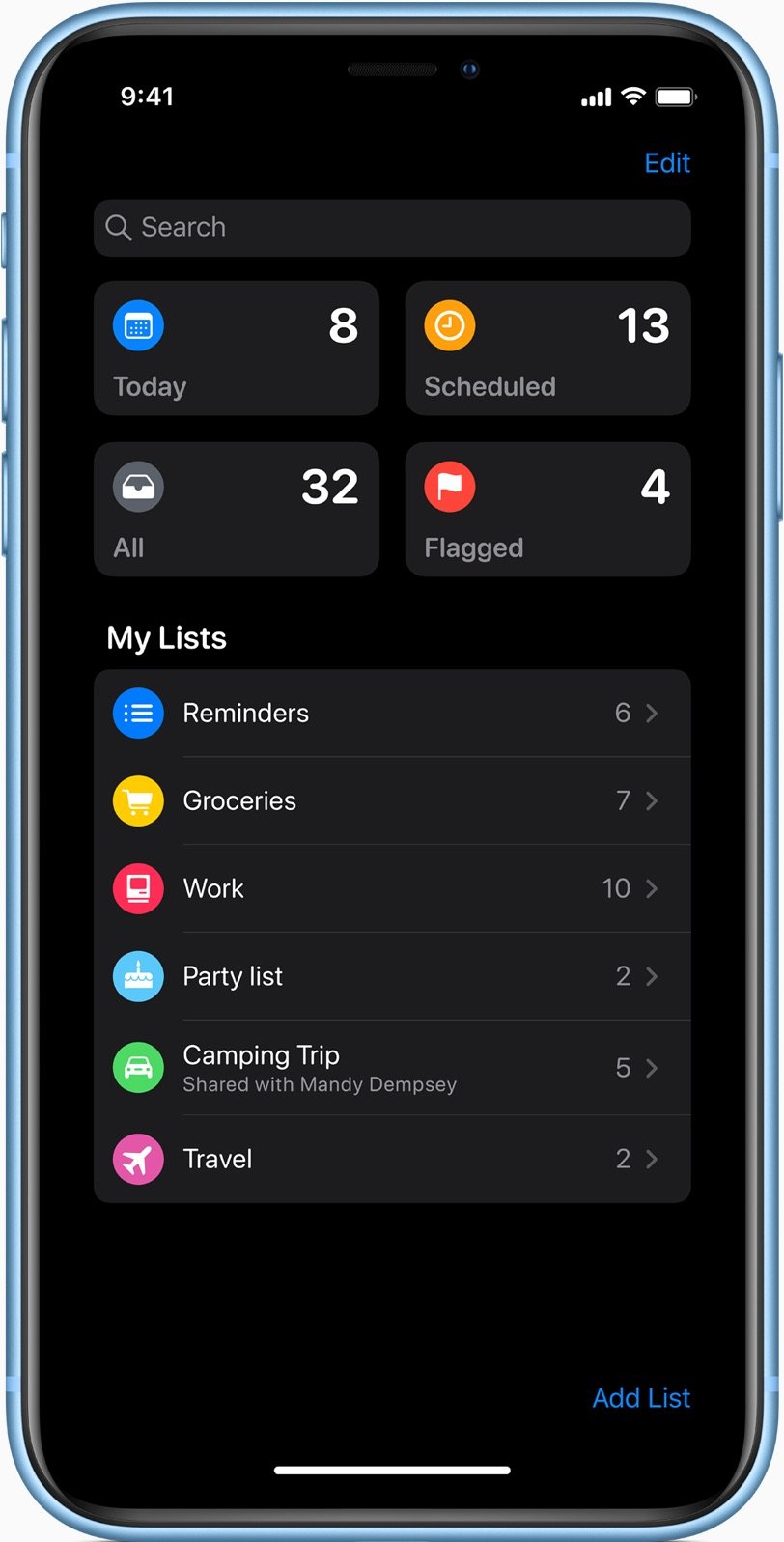This image features a blue Apple iPhone displayed prominently against a black background, indicating the phone is set to night mode. The screen is illuminated, revealing a comprehensive view of the "Reminders" app. At the very top, centered, a magnifying glass icon signifies the search function. To the top right, the "Edit" option is highlighted in blue.

Below these interface elements, the app showcases various reminders and their organizational tools. On the upper left, a small calendar icon corresponds with the label "Today," and adjacent to it on the right, the number "8" is displayed in a box, indicating eight specific reminders for the day. Towards the center top, another box labeled "13" suggests an upcoming date.

Moving down, the interface divides into categorically segmented boxes. The top left box, marked by a clock icon, reads "Scheduled" and shows the number "8" reminders. Directly beneath it, another box labeled "All" displays the number "32," accompanied by a small folder icon. At the bottom right of this section, the "Flagged" category is indicated, showing a red circle with a white flag and the number "4."

Below these sections, the "My List" category breaks into a vertical list naming different collections of reminders: "Reminders," "Groceries," "Work," "Party List," "Camping Trip," and "Travel." Adorning the bottom corner of the screen, the "Add List" option is vividly highlighted in blue, inviting users to create new reminder categories.

The phone's edges, colored in the blue finish of the device, subtly frame this intricate display of organization at your fingertips.